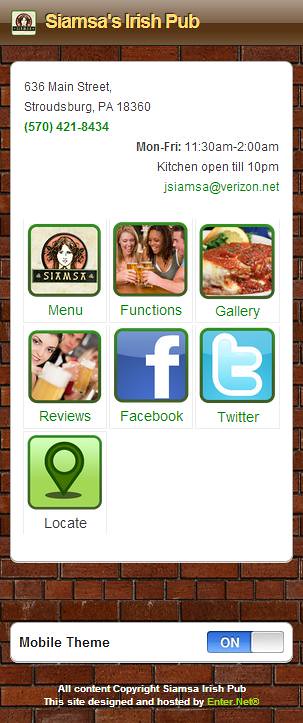This is a screenshot of a mobile website, likely taken on a phone. The background features a red brick texture. At the top, there's a brown gradient bar that reads "CM's Irish Pub," accompanied by a small logo on the left. Below it, a large white rectangular box displays the address: "638 Main Street, Stroudsburg, PA 18360," a phone number, "570-421-8434," and the hours of operation, stating the kitchen is open until 10 PM. An email address, "CMsPub@verizon.net," is also listed. Underneath this box are navigation buttons arranged in tiles: Menu, Functions, Gallery, Reviews, Facebook, Twitter, and Locate. At the very bottom, a toggle bar shows the mobile theme is switched on with an option to turn it off. Additionally, there's a note in small white text stating "All content copyright CM’s Irish Pub, site designed and hosted by Enter.net."